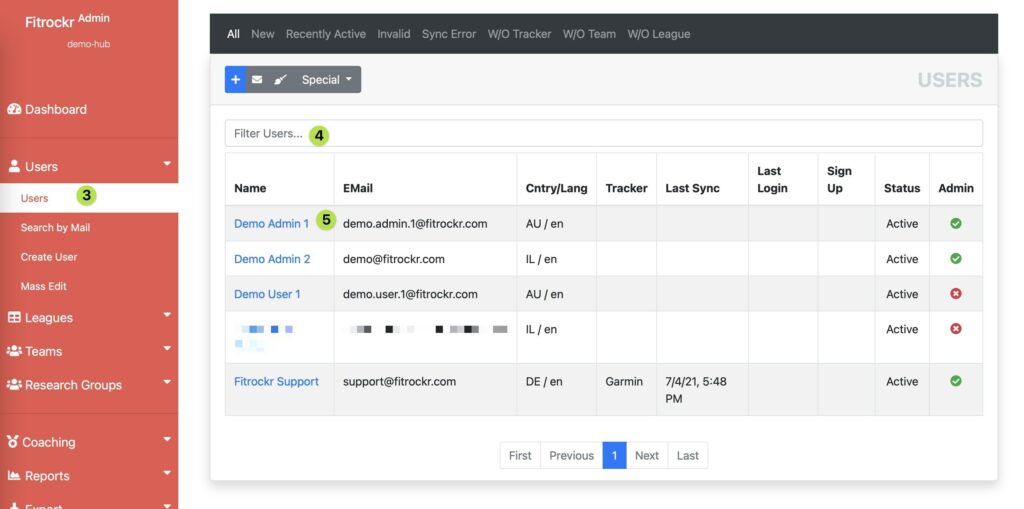This screenshot depicts a detailed demo hub of the FitRocker Admin page. The interface showcases a comprehensive dashboard, accessed via a vertical menu on the left, which is set against a light, rose-colored background. The menu items visible include Dashboard, Users (with the count of three displayed in a green circle), Users by Email, with a white line marking the boundary of this section across the width of the red menu, Search by Email, Create Users, Mass Edit, Leagues, Teams, Research Groups, Coaching Reports, and more items partially cut off from view.

Occupying about 80% of the right side of the screen, there is a blue-gray bar at the top featuring categories such as All, New, Recently Active, Invalid, Sync Error, Without Tracker, Without Team, and Without League. Below these categories, menu options and a plus button (indicative of adding new users) are present. Additional functions like Email, Graphic Editing, and Special (potentially color editing tools) are also below the blue bar. 

Filtering capabilities are represented by a filter for users (4). Further below, there are several columns titled Name, Email, Country, Language, Tracker, Last Sync, Last Login, Sign Up, Active, and Admin. The displayed data includes entries for 'demo admin one', 'demo admin two', and 'demo user one', along with a pixelated entry.

The information reveals their email addresses and countries (AU, IL), all in English. Despite the fields for Tracker, Last Sync, Last Login, and Sign Up being blank, the status for all mentioned users is Active. The Admin column distinguishes 'demo admin one' and 'demo admin two' with green checkmarks, while subsequent entries have red Xs in circles.

Finally, navigation buttons at the bottom of the screen indicate pagination controls with options for Previous, One, Next, Last, and a First button on the far left.